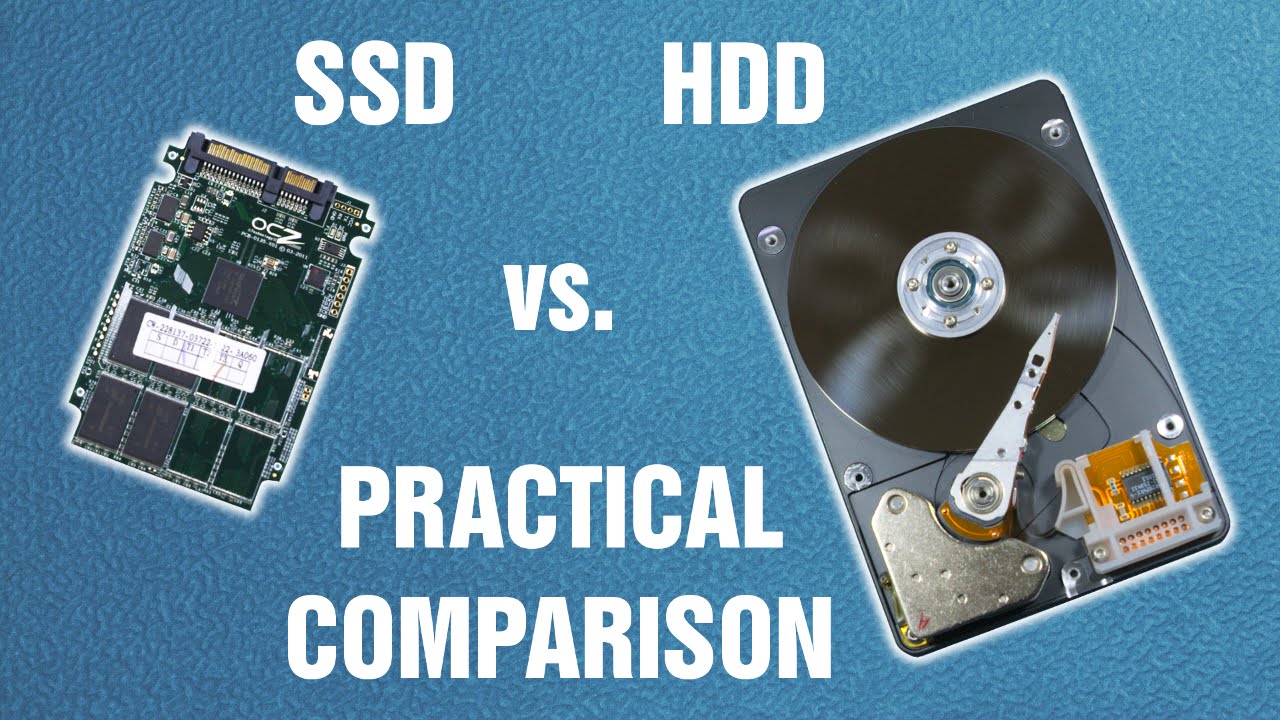The image is a detailed, comparative illustration of an HDD (Hard Disk Drive) and an SSD (Solid State Drive) against a blue speckled background. The title, "SSD versus HDD Practical Comparison," is written in white block-style print at the center. On the left, the internal workings of the SSD are displayed, showcasing four black solid-state chips and a small white node, emphasizing the absence of moving parts. On the right, the HDD reveals its mechanical components: a spinning platter, a magnetic recording head, an arm, springs, and a few control chips, resembling a mini record player. The image also highlights the size difference, with the HDD in a larger 3.5-inch case and the SSD in a smaller 2.5-inch case. White glowing lines accentuate the edges of each device, enhancing their visibility against the textured backdrop.